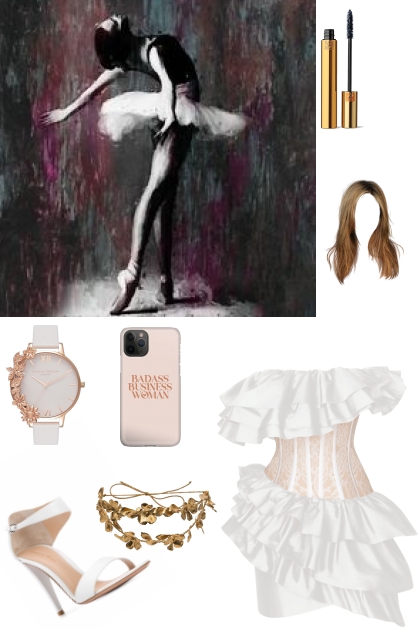This intricate collage centers around the theme of ballet and feminine elegance. Dominating the upper left is a vivid painting of a ballerina, illuminated as if by a spotlight. She stands gracefully on her tiptoes, arms elegantly arched behind her, head thrown back, gazing upward. Clad in a tutu, the ballerina's surroundings blend dark pink, green, and gray hues, enhancing the theatrical ambiance. Scattered around this art piece are various quintessentially feminine items: a pink and white corset, a sophisticated gold and white watch adorned with floral motifs on the left side, and a poised white high-heeled shoe. Nearby, a Grecian gold headband and lush blonde hair extensions and a wig contribute a touch of classic beauty. A tube of gold mascara adds to the makeup essentials present, accompanied by a phone case emblazoned with the bold phrase "badass businesswoman," reflecting confidence and modern flair. Additionally, an elegant white dress with gold sparkles and pleated ruffles sits gracefully at the bottom, tying the composition together with its delicate charm. This collection beautifully encapsulates the essence of ballet and feminine sophistication.